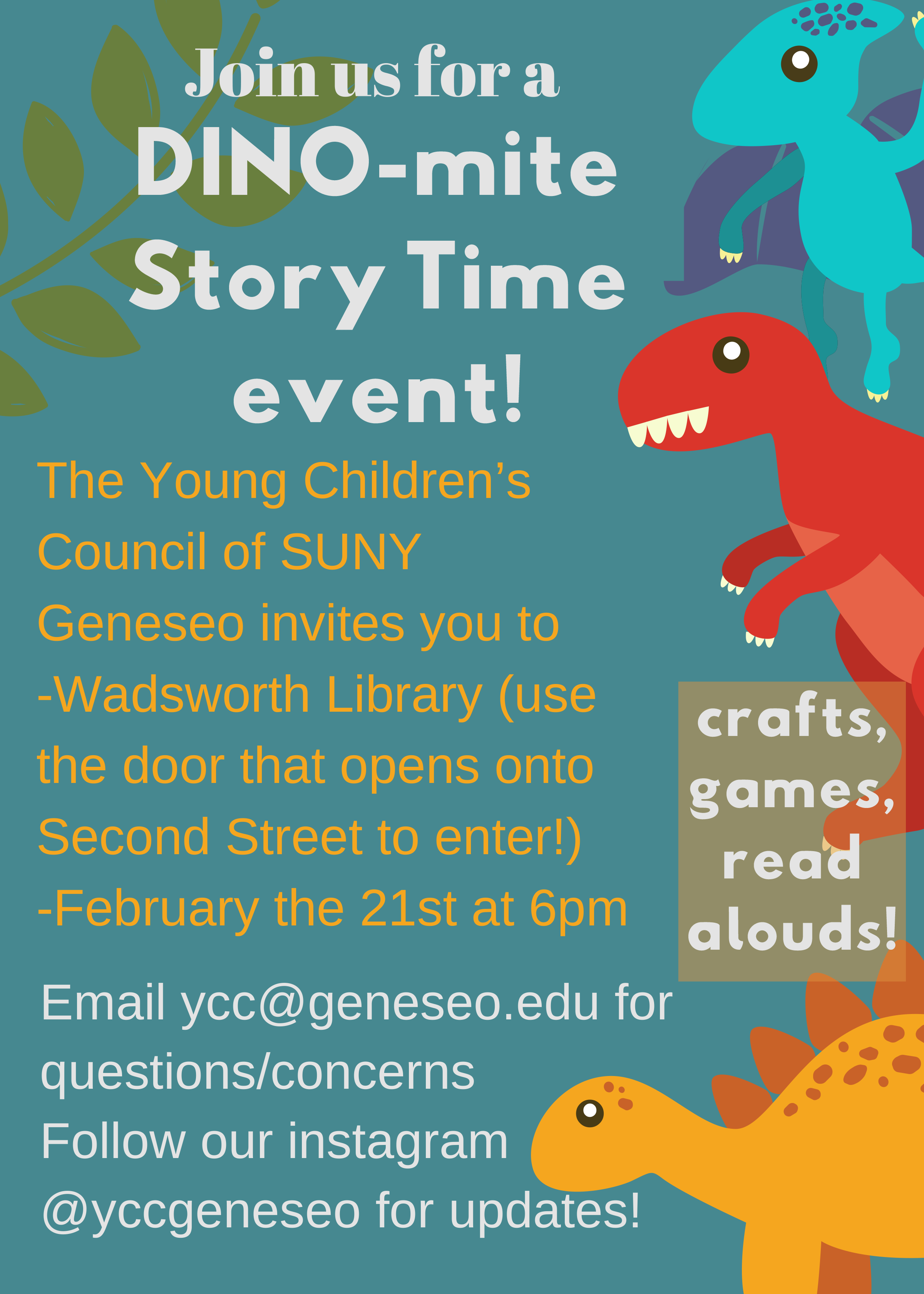This children's poster, with a blue background, invites kids and their families to a Dino-Mite Storytime event hosted by the Young Children's Council of SUNY Geneseo at Wadsworth Library. The right-hand side features adorable, friendly cartoon dinosaurs, with one blue, one red, and one orange, all illustrated in a non-threatening, childlike style. Decorative elements include a green leaf vine on the left. The top text, written in white, reads, "Join us for a Dino-Mite Storytime Event," while the central text, in yellow, states the hosting details and the venue using the door on 2nd Street. The event is scheduled for February 21st at 6 p.m., where activities will include crafts, games, and read-alouds. For questions or concerns, attendees are encouraged to email ycc@geneseo.edu. Additionally, updates are available by following @yccgeneseo on Instagram.